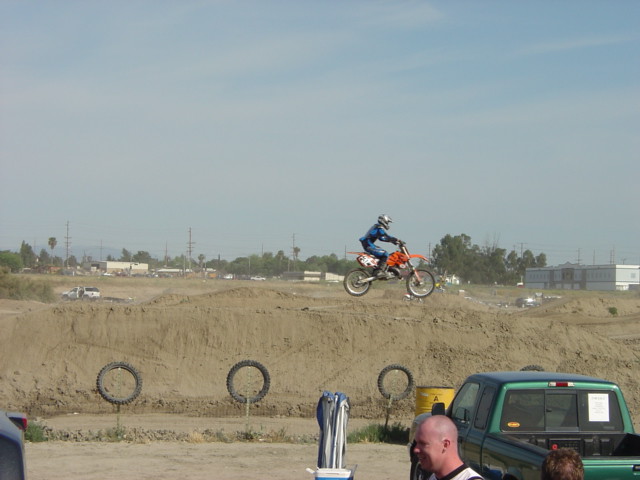The photograph captures an outdoor dirt bike course carved into the side of a hill, featuring a high-adrenaline motorcycle stunt. A rider clad in a blue and black uniform, with black boots and a silver helmet, soars through the air on an orange and white motorcycle, mid-jump over a series of hoops or tires. The dirt ground below, primarily brown and covered in soil, accentuates the ruggedness of the setting. In the foreground, a green pickup truck is visible, with various onlookers around it, including one person standing behind and another to the side of the truck, whose profile is discernible. The horizon reveals trees and industrial buildings, all set under a clear blue daytime sky, framing the scene of this extreme sport event.